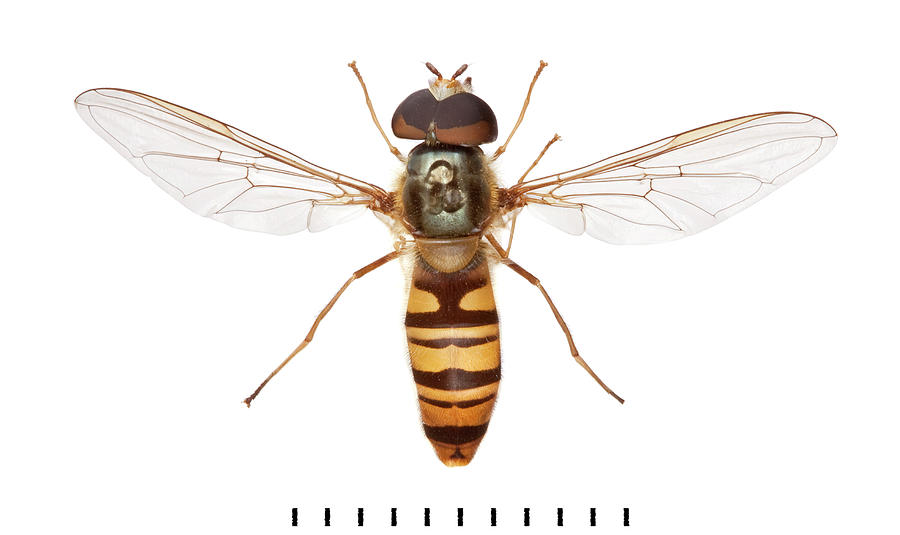This detailed illustration showcases an insect, likely a bee, hornet, or wasp, viewed from above. The body features alternating stripes of brown and yellow, pointing towards the bottom of the frame, with its distinctly veined, transparent wings spread wide. The head, resembling a semi-oval shape in a deep brown hue, leads into a grayish or grayish-brown thorax. Extending from its body are six legs—two forward-facing, and the rear legs splayed out at a 45-degree angle. The background is a stark white, highlighting the intricate detailing of the insect, including its antennae and the series of 11 solid black hash marks below it.